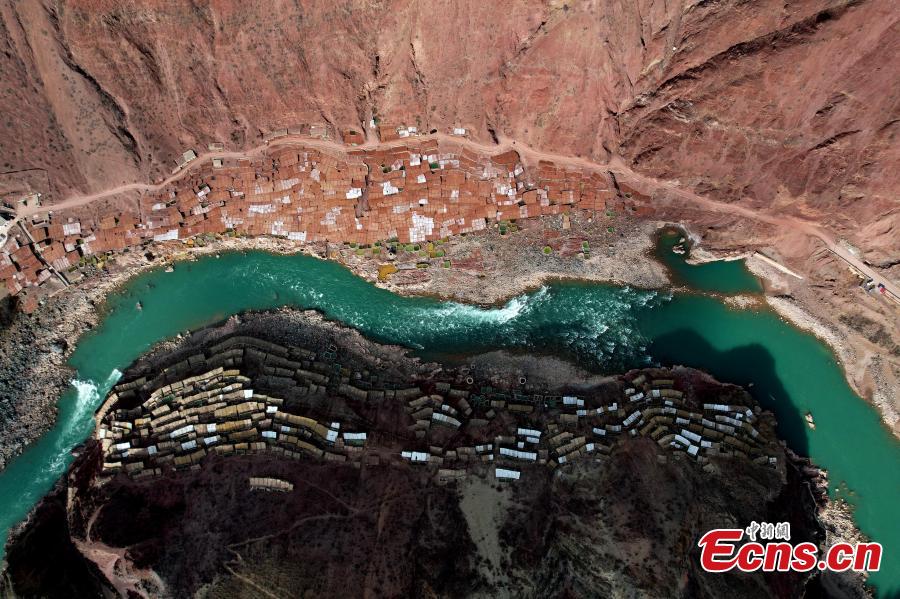A photorealistic aerial view showcases a vibrant green river winding through a rugged landscape of red cliffs and rocky formations. The river, interspersed with sections of white water rapids, arcs through the image, starting from the lower right, curving leftwards midway, and descending to the lower left. Above the river, the top portion of the image features a sunlit red cliff, with the lighter-hued mountains framing the scene. Beneath these cliffs lie a series of reddish-colored squares, potentially buildings or other structures, indicating a populated area nestled against the natural rock face. The left side displays a zigzagging road running parallel to the river. The lower sections of the rocky terrain, now shrouded in shadow, contrast starkly with the sun-drenched cliffs above. In the bottom right corner, the image includes the text "ECNS.CN" in red font, outlined in white, accompanied by three stylized characters, likely of Chinese origin.